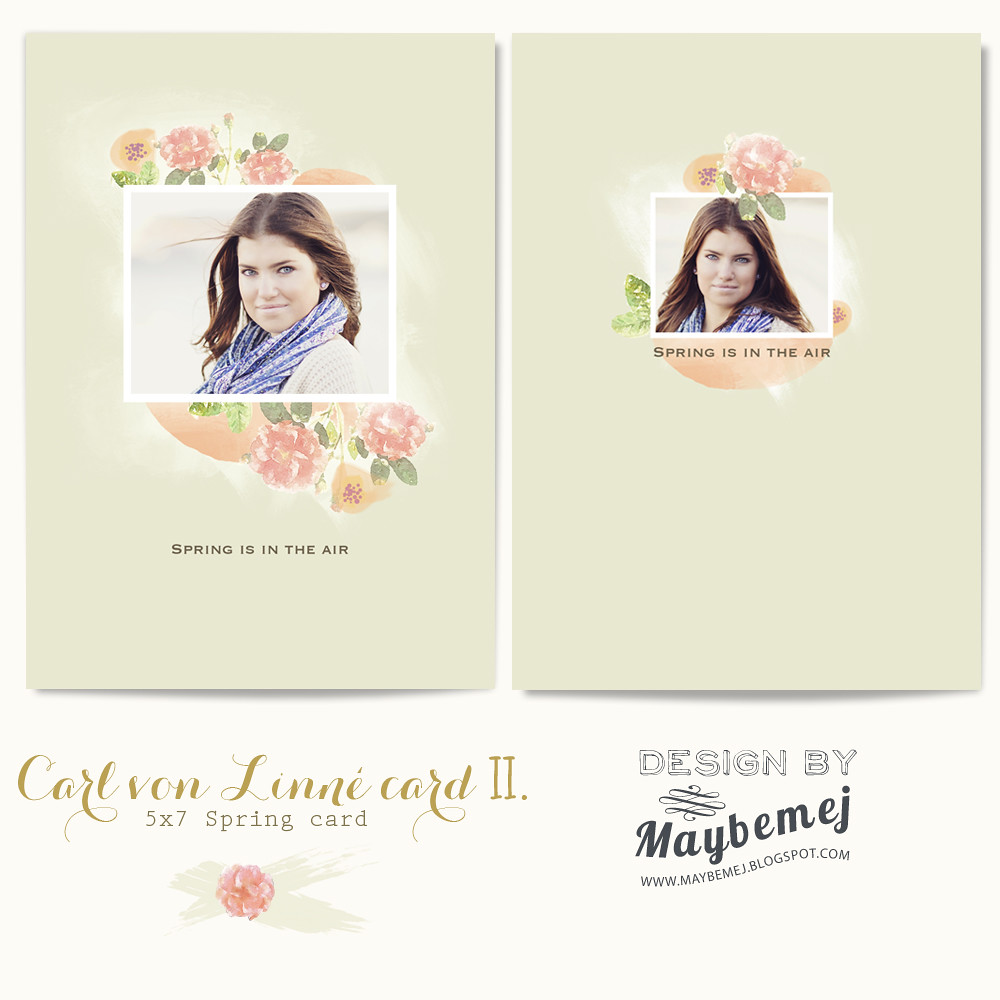The advertisement showcases a set of 5x7 inch greeting cards centered around the theme "Spring is in the Air," designed by Maybemej.blogspot.com. Each card features a young woman in her 20s with dark brown hair and light-colored eyes, adorned with shiny, possibly diamond earrings. She exudes a soft smile without showing her teeth and is dressed in a white cardigan, complemented by a blue and white scarf. Her hair appears to be gently blowing in the wind. 

Both cards display her in slightly different poses and are bordered by vibrant floral graphics. The card on the left has her picture in the middle with surrounding pink flowers, whereas the card on the right has her image with a pink flower drawn on top. The background of the cards is a light green color. Each image is enclosed within a white border and features the text "Spring is in the Air" in polished font. Below the central images, in gold text, it reads "Carl Von Linn Card II 5x7 Spring Card". The bottom right of the display holds a small graphic with the designer's moniker and the URL, "Designed by Maybemej.blogspot.com".